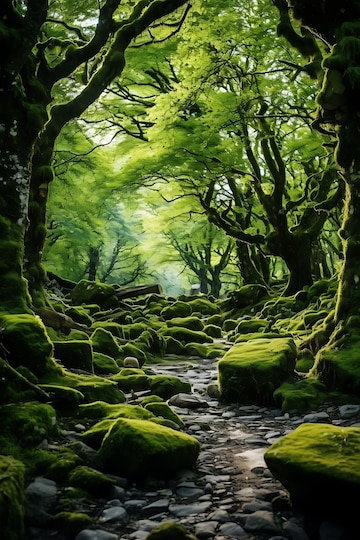The image depicts a surreal, CGI-generated scene of a stream bed winding through a forest, festooned with gray rocks and minimal water flow. The stream curves around uniformly moss-covered outcroppings on the shore, with a lush covering of moss extending up to the bases of towering deciduous trees flanking the scene. The trees, adorned with vibrant green leaves, form a dense canopy overhead, allowing only slivers of natural light to penetrate, creating an almost shaded, tunnel-like effect along the path of the stream. In the distance, the canopy opens slightly, revealing hints of sunlight and the next hill, suggesting an expansive, yet hidden landscape beyond the immediate view.